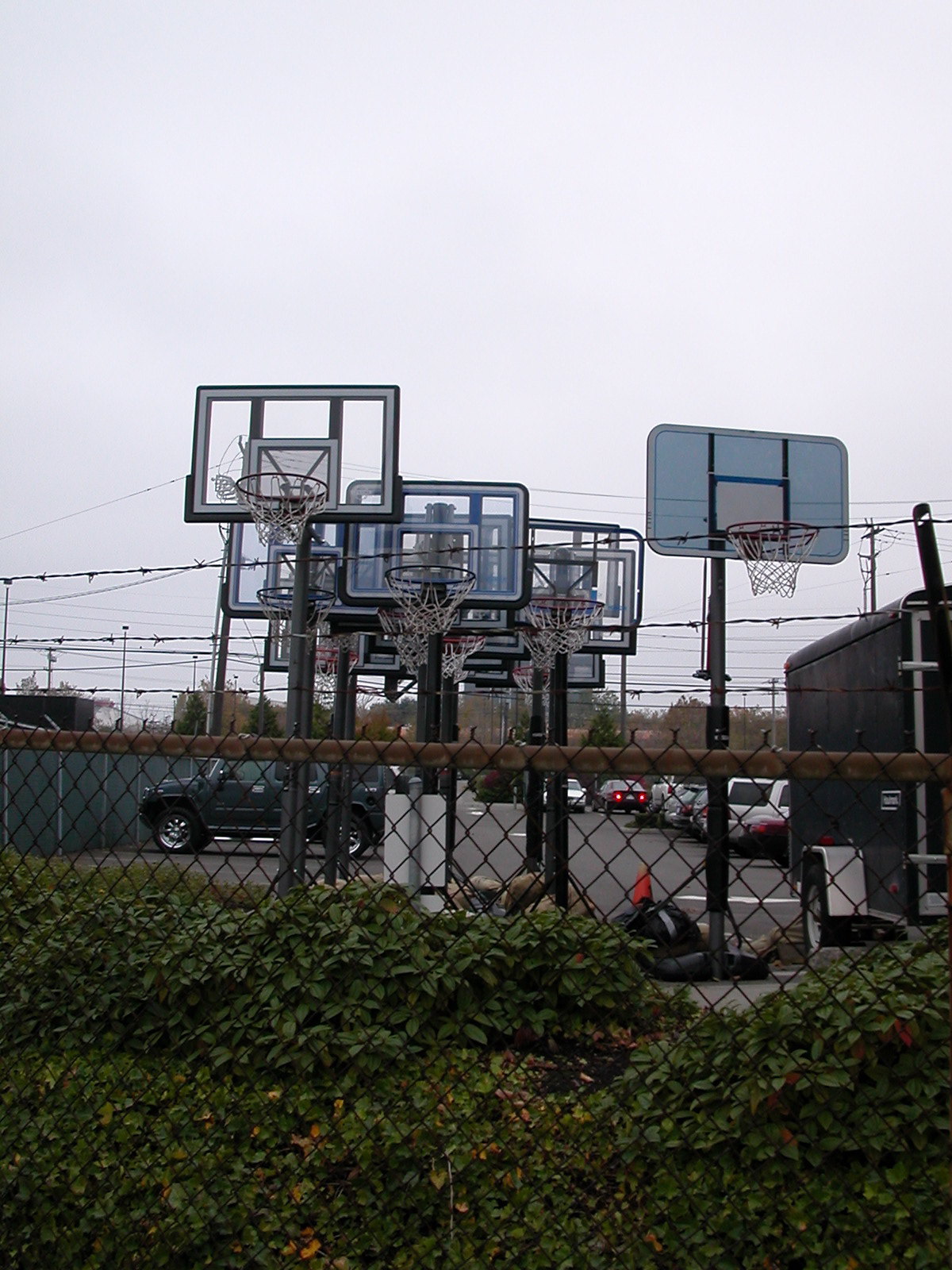The photograph depicts a gray sky hovering over a parking lot filled with a variety of cars, framed by a rusted metal fence topped with barbed wire. Green shrubbery encroaches the base of the fence, adding a touch of greenery to the scene. Beyond the fence, about ten tall, portable basketball hoops stand prominently, each equipped with clear backboards and white nets, all facing towards the viewer. The hoops appear neatly arranged, ready for a game, yet separated by the fence barrier. On the right side of the image, a small black trailer is noticeably parked near the basketball hoops. The entire composition captures the hoops, cars, and overcast sky, creating a detailed, multi-layered image.